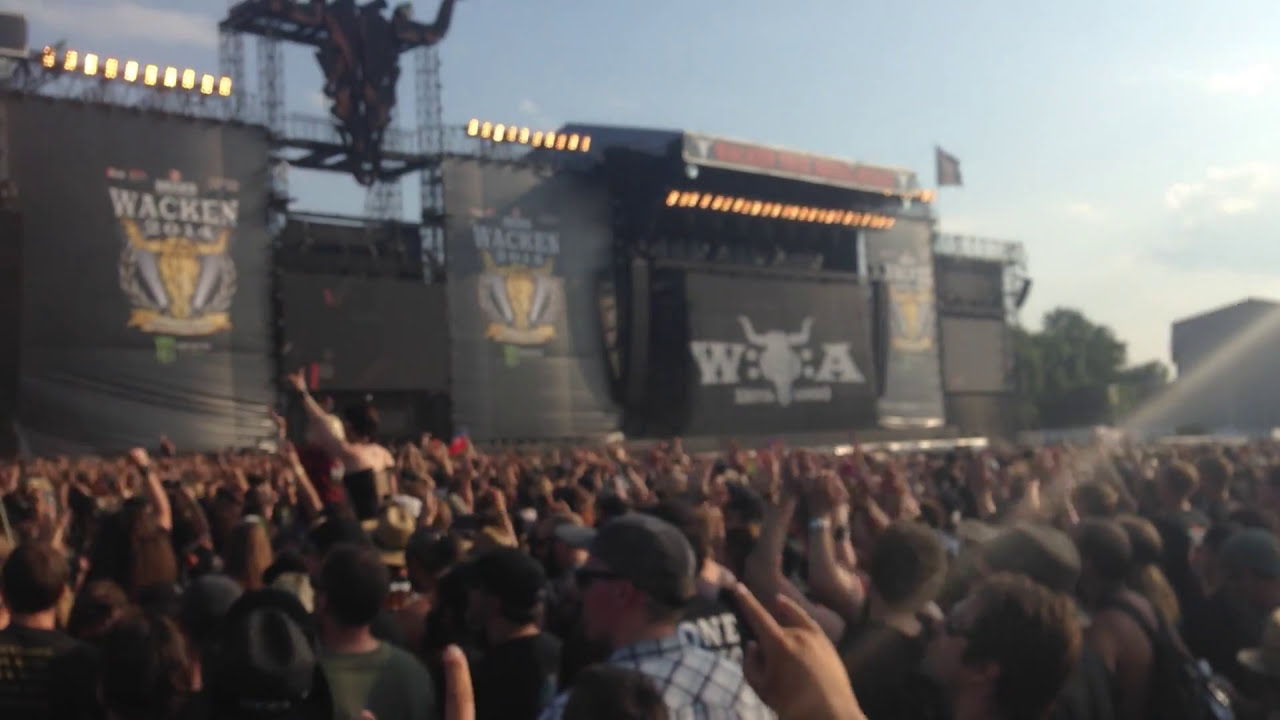A vibrant outdoor concert scene is captured with a massive crowd of people closely packed together, many wearing hats and some women perched on shoulders, all facing towards a large stage on the left. The stage is adorned with several banners emblazoned with the text "WACKEN 2014" and a distinctive yellow bull's head logo encircled in white. The banners are hung on black material stretched between metal scaffolding, which extends high into the sky. Above the banners, there are rows of bright yellow and orange lights. Dominating the center stage is a large banner with a white background displaying the letters "W" and "A" flanking a central bull emblem. The upper right of the image reveals a bit of blue sky with sunlight streaming through, casting reflections onto the crowd. In this section, a densely leafed dark tree and a light grey building with a sloped roof can also be seen, adding to the bustling yet scenic atmosphere of the event.